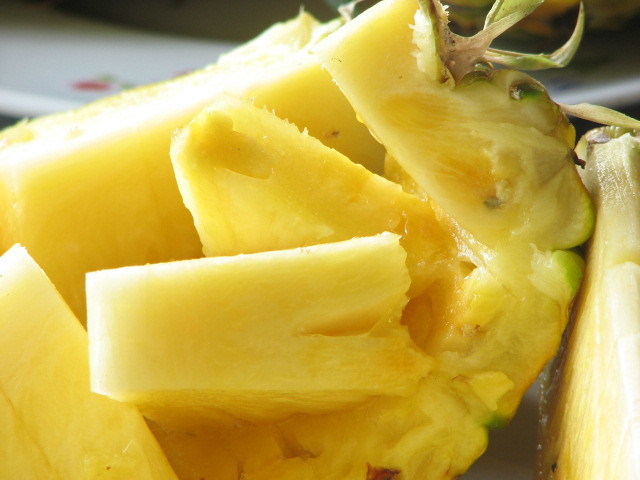This close-up image captures a primarily sliced, fresh pineapple resting on a table indoors. The pineapple is predominantly an orangish-yellow color, with some green leaves still attached to the stem, visible in the top right. While several triangular wedges have been cut from the fruit, some pieces remain uncut, and the fruit's thick interior is evident. On the right, a section of the pineapple's mass leans against a white piece of the fruit. The background features a table with a blurry cherry or cherry design in the upper left. Additionally, there’s a faint, out-of-focus white object in the upper right, possibly a plate, adding to the overall indoor setting.